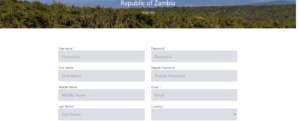This image appears to be a highly minimized and unclear screenshot of a website's interface. The main content area has a white background, featuring two columns of four grey rectangular sections, making a total of eight blocks. Above each grey block is a heading, and all but one block contain text, which is indistinct due to the image size. Specifically, the grey blocks on the left column contain one-word entries in the first two blocks, possibly two words in the third, and one word in the fourth. The right column has one-word entries in the top three blocks, while the last block is empty, featuring only its heading. The banner at the top of the site appears to depict a forest scene with unreadable white text in the center. The clarity of the image is severely restricted, making it challenging to discern detailed content within the blocks or the banner.